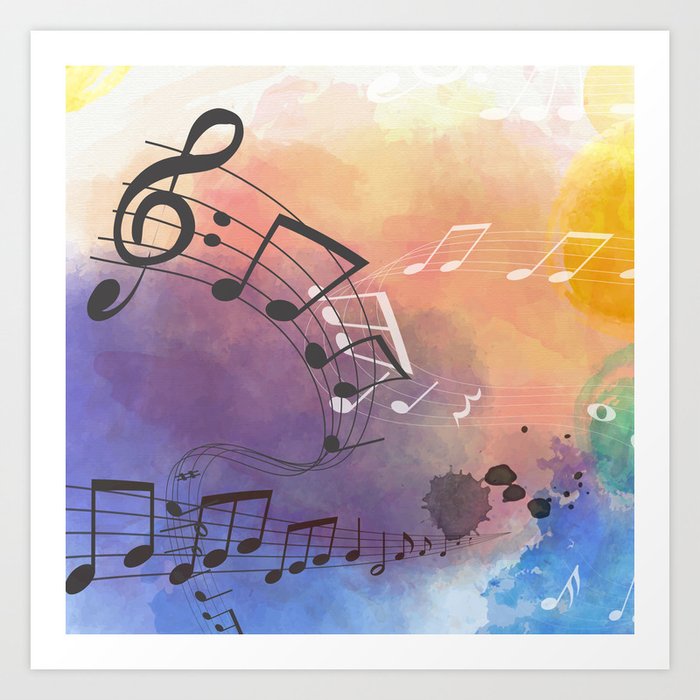The image showcases an abstract watercolor painting with a vibrant and dynamic blend of colors, including yellow, pink, peach, tan, cyan, blue, green, purple, and red. The swirled watercolor background creates a richly stained effect, almost resembling colorful clouds. Dominating the composition are several musical scales that wind through the image like ribbons. From the top left, bold black music notes curve down toward the bottom left corner. Meanwhile, another set of white music notes swirls from the middle right, wrapping around to the center and then to the bottom right. Additionally, more black notes cascade from the top left down toward the lower edge of the painting. The artwork is framed with a white mat, set against a lilac-gray background, creating an elegant presentation that celebrates the vibrant and dynamic interplay of music and color.